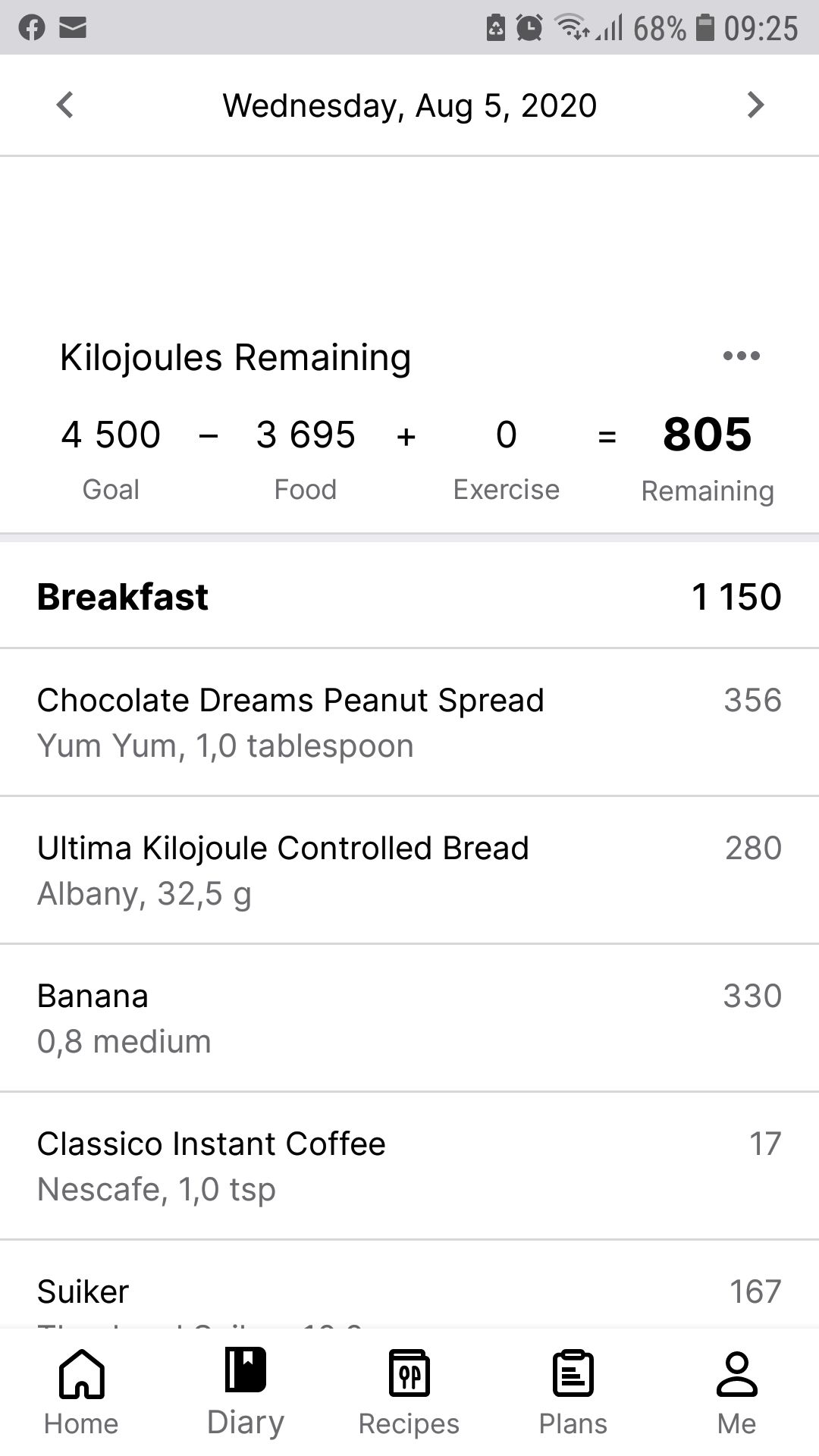This detailed black and white iPhone screenshot, taken at 9:25 AM with 68% battery, displays a nutrition tracking app on Wednesday, August 5th, 2020. The interface shows icons for Facebook and email in the status bar. At the top of the screen, it reads "Kilojoules remaining," with three dots to the right indicating additional options. Below, calculations for daily kilojoule intake are shown: 4500 - 3695 + 0, equating to 805 remaining, categorized into goal, food, and exercise.

For breakfast, the detailed listing includes:
- Chocolate dreams peanut spread, 1 tablespoon: $3.56
- Ultima kilojoule controlled bread: $2.80 for 2 slices (205 grams)
- Banana, 8 medium: $3.30 each
- Classico instant coffee, 1 tablespoon: $17.00
- Nescafe with suiker (sugar): $1.67

At the bottom of the screen, navigation options are displayed: Home, Diary, Recipes, Plans, and Me. The entire interface is monochromatic, hinting at a potentially foreign localization due to distinct formatting of numbers and currency.